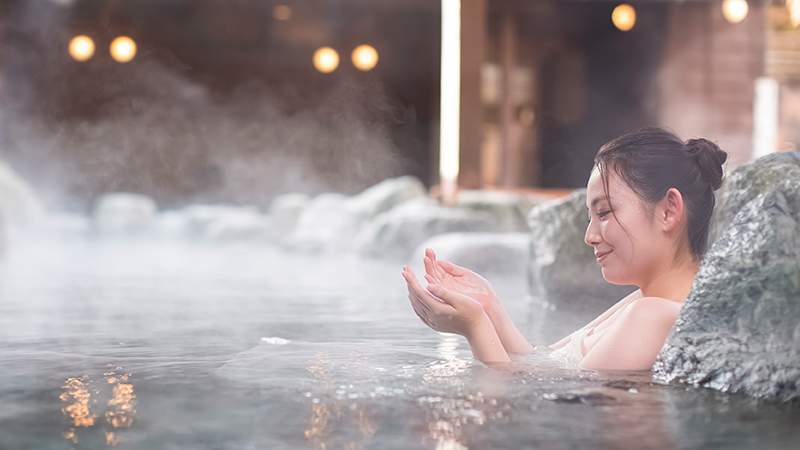In this atmospheric indoor photograph, an Asian woman is relaxing in a spa, immersed in a hot tub up to her shoulders. Leaning against a porous, gray rock on her right side, she smiles serenely down at her upturned palms, enjoying the sensation of water dripping off them. Her long dark hair is pulled back into a bun, with a few wet strands hanging loose over her face. The water around her is light gray, reflecting the ambient light, further enhancing the tranquil setting. Steam rises from the hot water, creating a misty effect that shrouds the background, where blurry, irregularly shaped rocks and walls embedded with soft, out-of-focus yellow and orange lights add a warm glow to the scene. The overall ambiance is peaceful and serene, capturing a moment of pure relaxation.